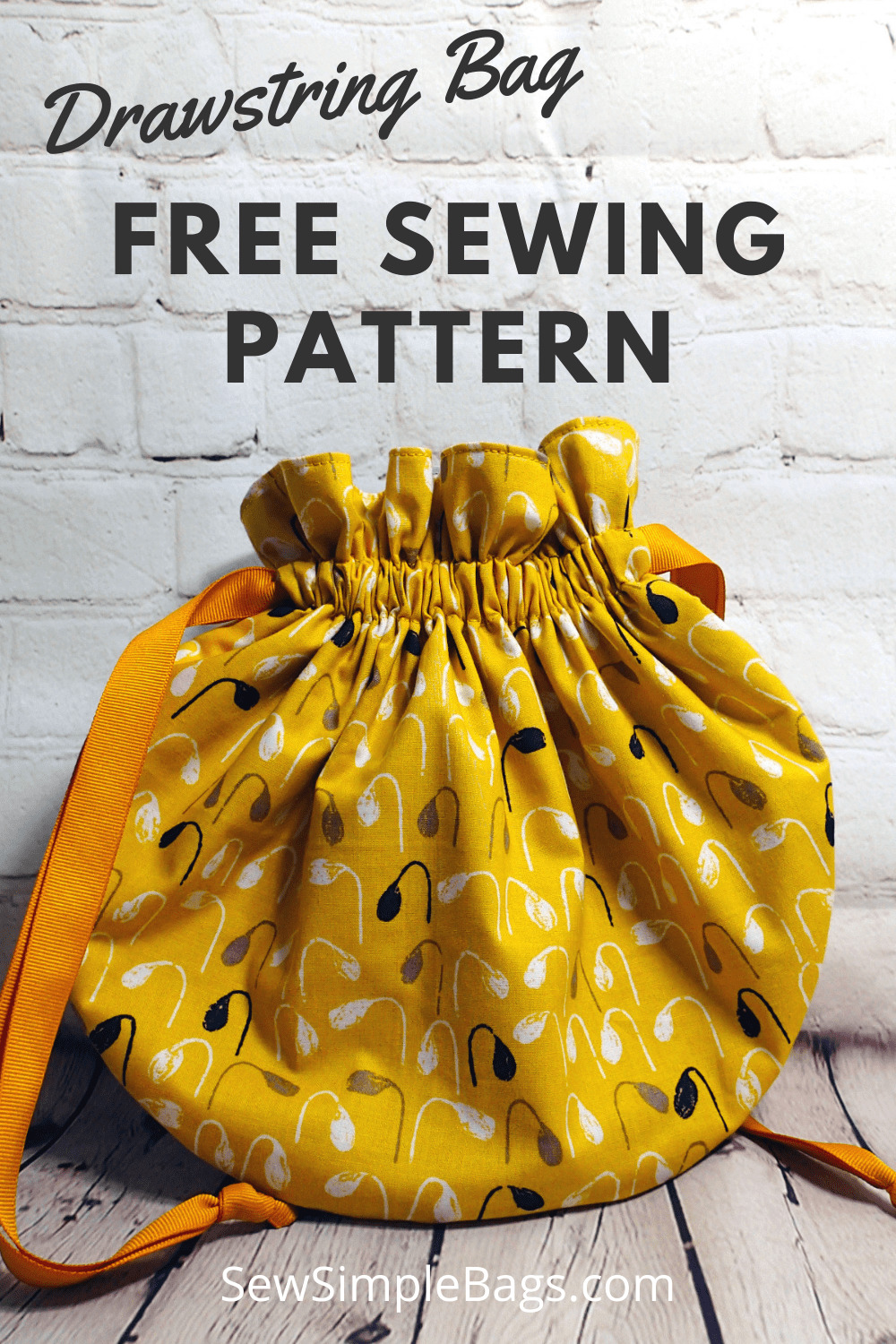The image is an advertisement for a free sewing pattern from soosimplebags.com. It features a prominently displayed yellow drawstring bag adorned with a decorative pattern consisting of black, white, and gray teardrop shapes with lines, reminiscent of small olives or buds. The bag includes yellow drawstrings used for closure and additional straps for carrying. The background showcases the bag lying on an old wooden floor with a rustic, white-painted brick wall behind it. Text above the bag reads "free sewing pattern" in a clear font, with "drawstring bag" written in cursive above it.